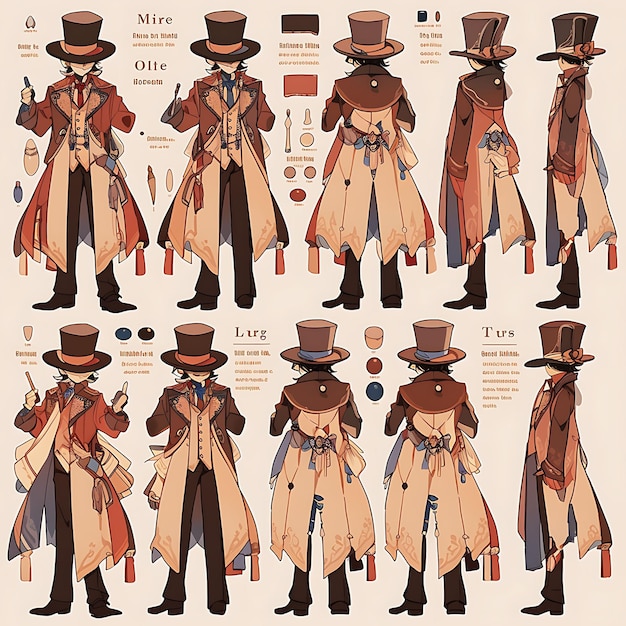The image is a detailed artist's drawing of a young man dressed in a dapper outfit, depicted in ten different poses. The man sports a bowler hat, adorned with what appears to be a feather on the right, which complements his suit. He is clothed in a dark brown to light brown long coat that reaches his knees, notable for its many pockets and attachments, suggesting a cleverly designed jacket suited for concealment. His ensemble includes a vest, a red tie, green pants, and dark boots. 

The image portrays the man in various angles: directly facing forward, showing his entire back, profile views, and intermediate angles. In some frames, he is holding different items or has his hands in his pockets, while in others, his arms are raised. He also carries a beige book bag with a brown flap, inscribed with some text that appears to be in an unrecognized language. The consistent details across the drawings, like his top hat and coat with multiple pockets, suggest a character with a sense of mystery and a clever, perhaps mischievous, demeanor.